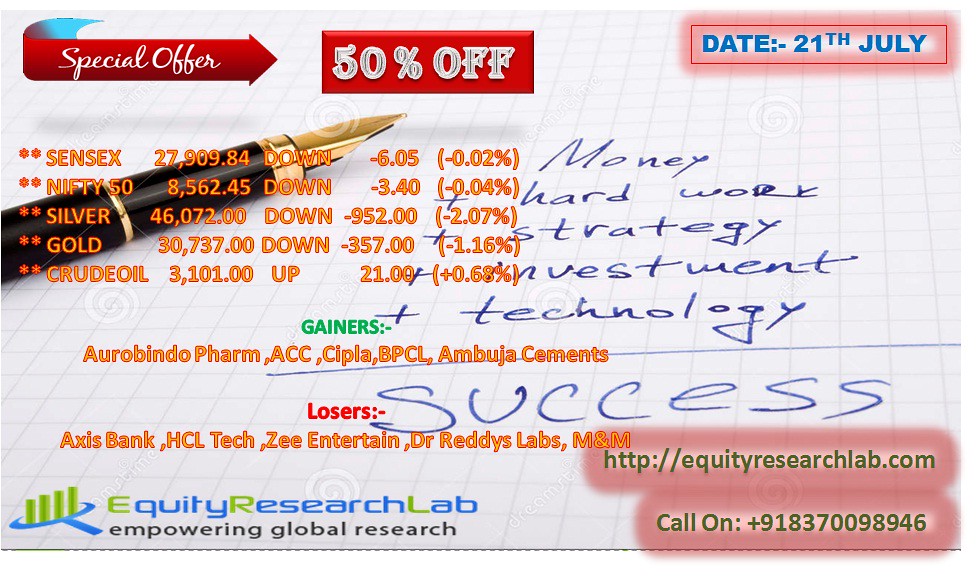This advertisement features a special offer prominently in the upper left corner, with a red arrow pointing right towards a "50% off" promotion. In the upper right corner, the date "July 21st" is displayed in blue. Below this, a gold pen rests on a piece of graph paper with blue writing that reads, "money, hard work, strategy, investment, and technology equals success," suggesting a financial seminar promotion. The advertisement provides detailed information on various financial metrics, including a reference to "Sensex" at 27,909.84, down by 6.05 (-0.02%). It also lists commodities such as silver, gold, and crude oil with their respective price changes, alongside gainers like ACC and CIPLA and losers such as Axis Bank and HCL Tech. The bottom left of the page features "Equity Research Lab" in blue and green lettering, accompanied by the tagline "empowering global research." To the right, within a pink box, the website "equityresearchlab.com" is provided, along with additional contact details including an email address and phone number.